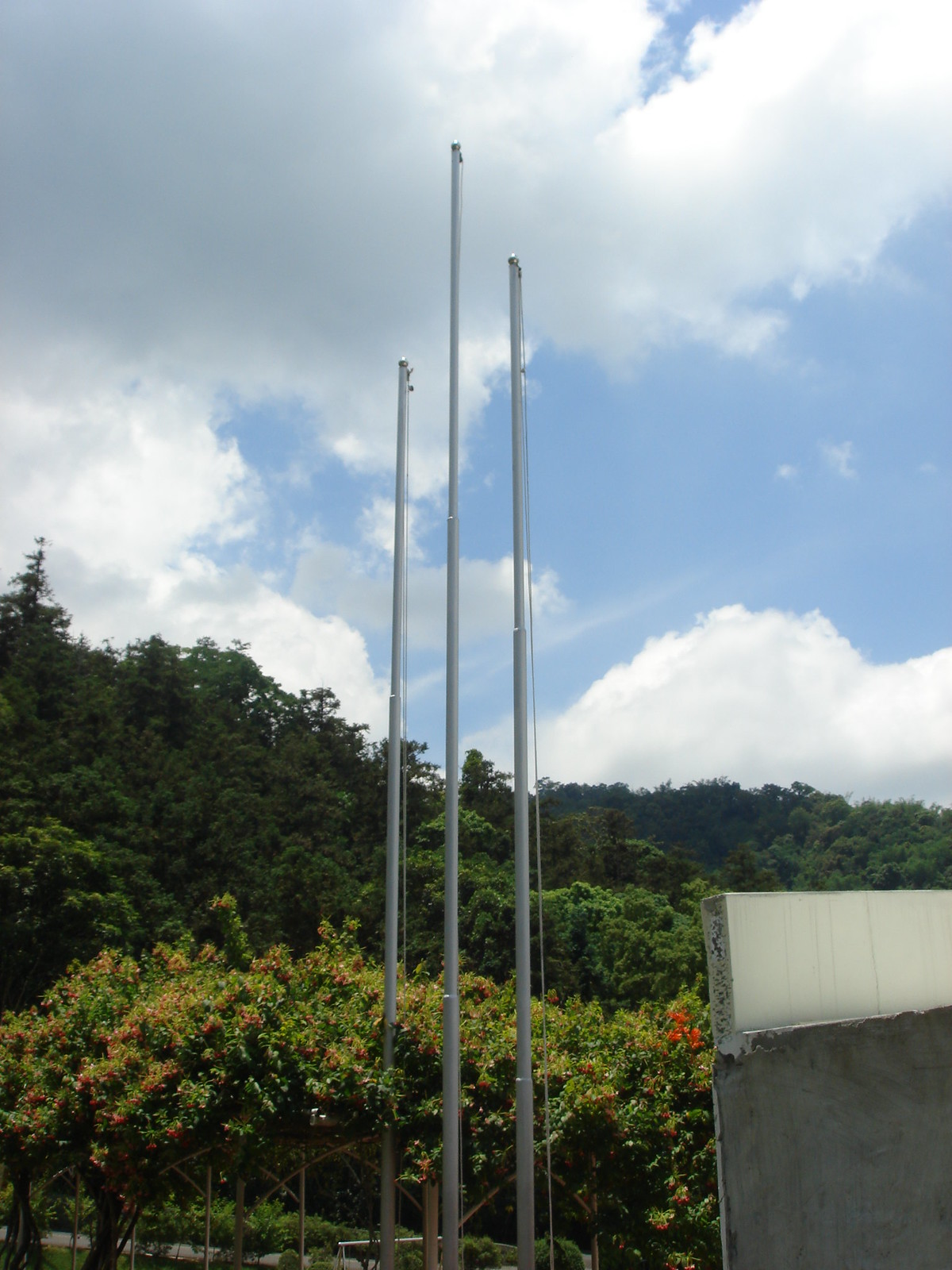This outdoor scene captures three stainless steel flagpoles of varying heights standing against a backdrop of dense greenery. The tallest flagpole is in the center, flanked by progressively shorter ones on either side. The flagpoles have white ropes but no flags and rise into a bright blue sky filled with puffy white and gray clouds, suggesting impending rain. Behind the flagpoles, a lush hill or small mountain is covered in evergreen trees. Closer to the camera, there are flowering trees with red buds and blossoms. On the right side of the image, a concrete wall with a white streak can be seen. Additionally, a path leads to a bench near the flagpoles, enhancing the serene and picturesque ambiance of this landscape.